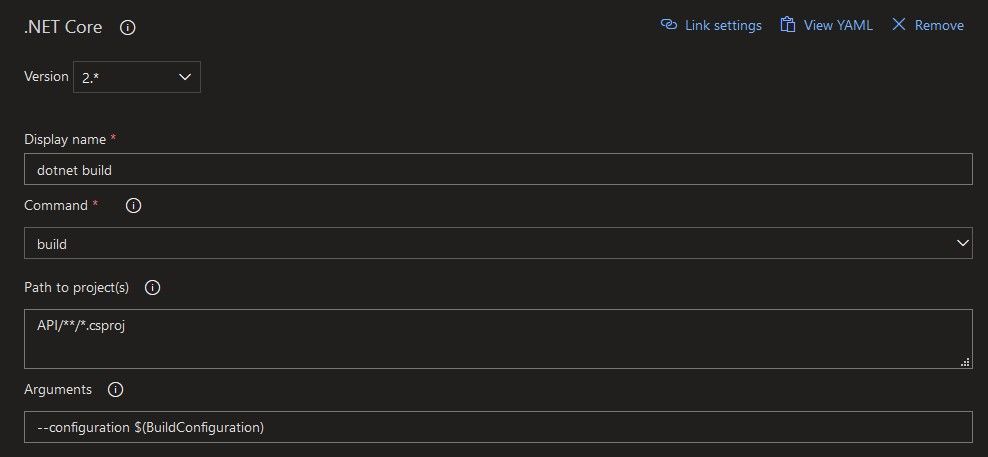The screenshot depicts a .NET Core configuration interface set against a black background. At the top, navigational options such as "link settings," "view YAML," and "remove" are visible. The version is displayed as "2," and the "display name" field is highlighted with a red asterisk, indicating it is a required field. Inside this box, the text ".NET Build" is entered. 

Further down, another section marked "command" also features a red asterisk, signifying it as mandatory. Within this input box, the word "build" is entered, accompanied on the right by a downward arrow indicating a dropdown menu. Below this, the label "path to projects" appears, along with an information icon (indicated by an “i” in a circle). The corresponding input box contains the path "api/**/*.*proj."

To the far right of the path input box, there is a sequence of three icons resembling bar graphs: one single square, another with two squares stacked vertically, and a third with three squares stacked. 

The last section is labeled "arguments" and also features an information icon. The input box here contains the text "--configuration $(BuildConfiguration)," with both "Build" and "Configuration" capitalized and concatenated into one word.